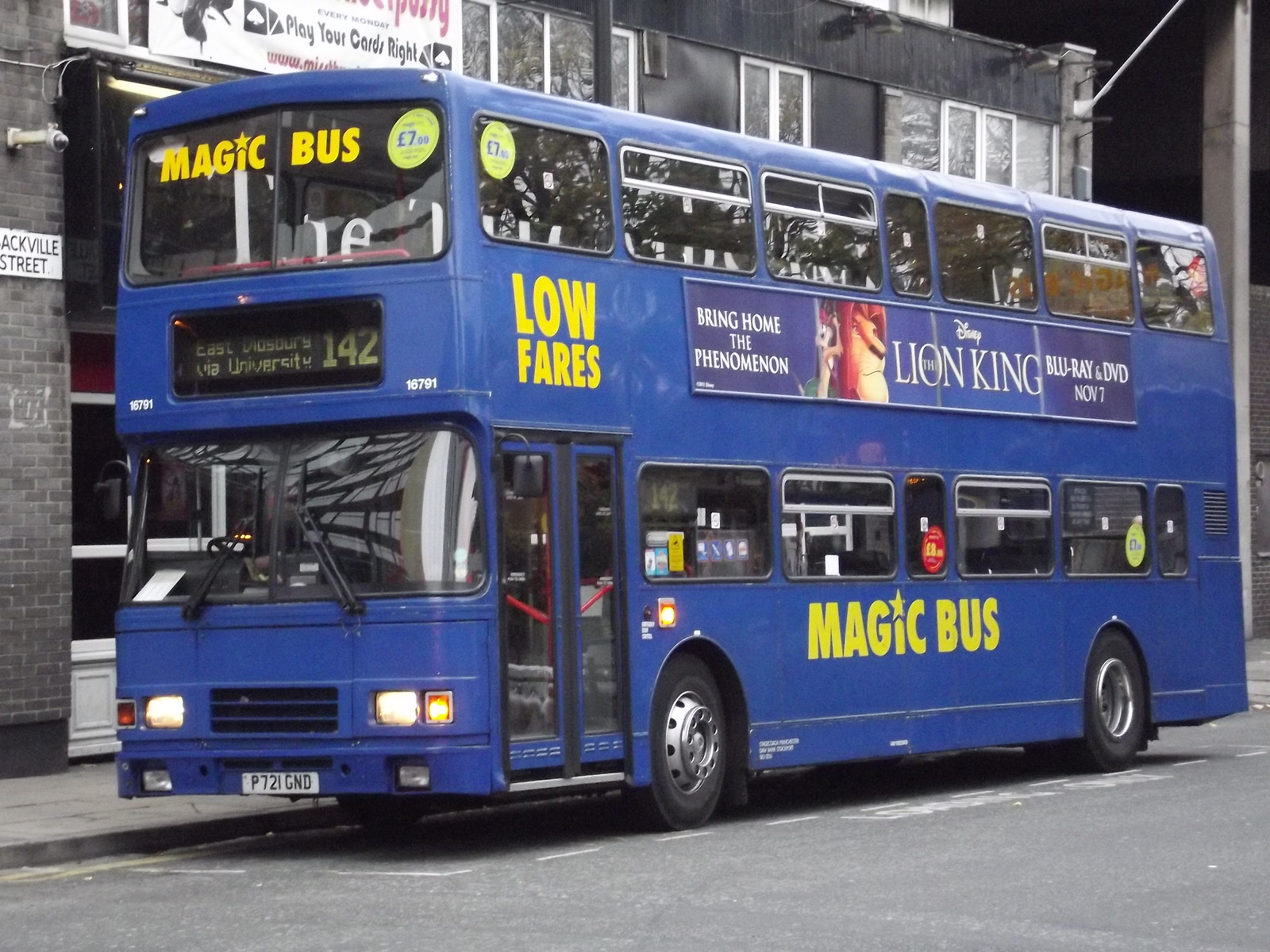This image features a blue double-decker bus prominently positioned in the center, moving from right to left. The bus displays several eye-catching elements, starting with "Magic Bus" written in yellow text on both the side and the windscreen of the upper deck, where the 'i' is uniquely dotted with a star. Below the windows of the upper deck, more yellow text reads "Low Fares." A large advertisement for Disney's The Lion King is plastered between the upper and lower halves of the bus. Above the driver's windshield, the words "East via University" are visible, along with the route number 142. The bus, currently stationary by the side of the road, features a front license plate, headlights, and black wheels clearly visible against the street below. In the background, there is a gray building, adding urban context to the scene.